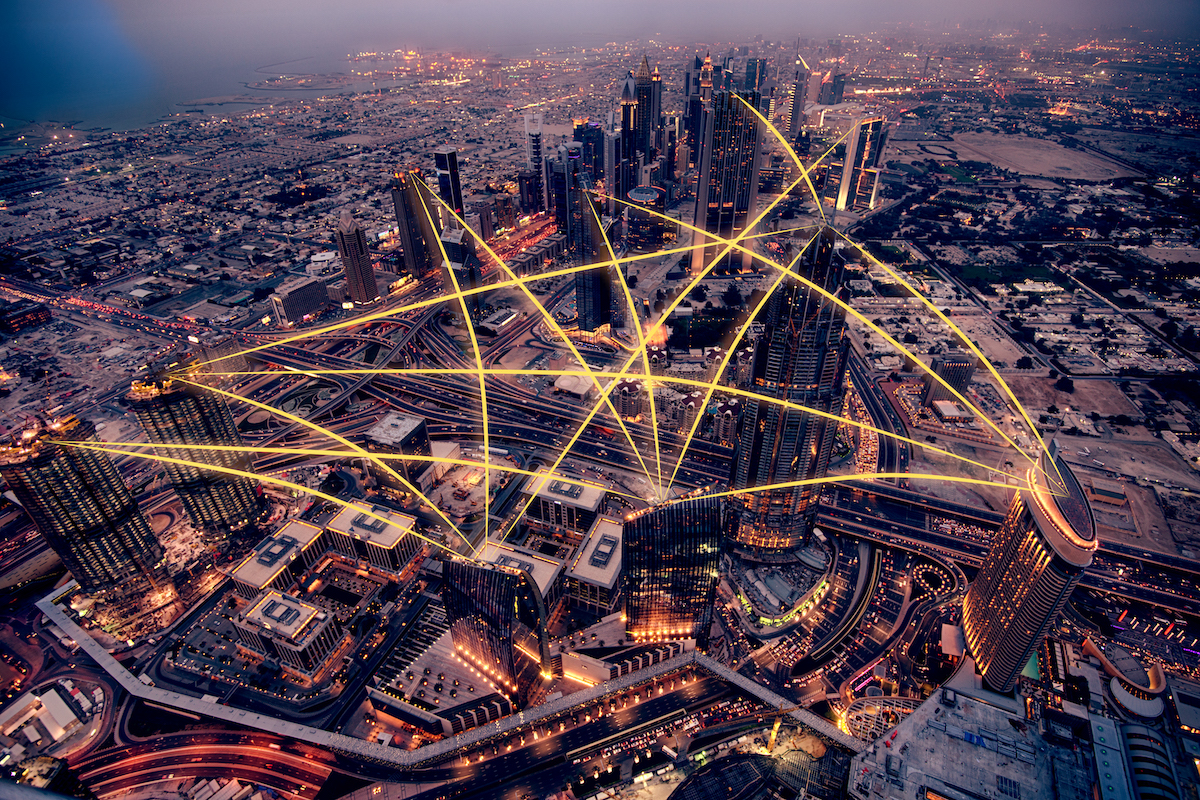This aerial image captures a bustling cityscape at dusk, viewed from high above as if from an airplane or drone. The city is dotted with numerous skyscrapers and tall buildings concentrated in the center, tapering off to shorter structures towards the edges. The urban expanse is bisected by large highways and possibly a railway system visible through the middle.

Prominent in the scene is a network of bright yellow lines stretching between the tallest buildings, creating a striking web-like pattern. These lines, which resemble a communication network or hub system, artistically connect the buildings, emphasizing a sense of connectivity. The city lights are on, illuminating the scene with a warm glow against the dim twilight backdrop of greys and darker tones. In the distance, towards the edge of the image, water is faintly visible, suggesting the city’s proximity to a lake or waterfront. The image overall exudes a dynamic, interconnected urban environment transitioning into night.